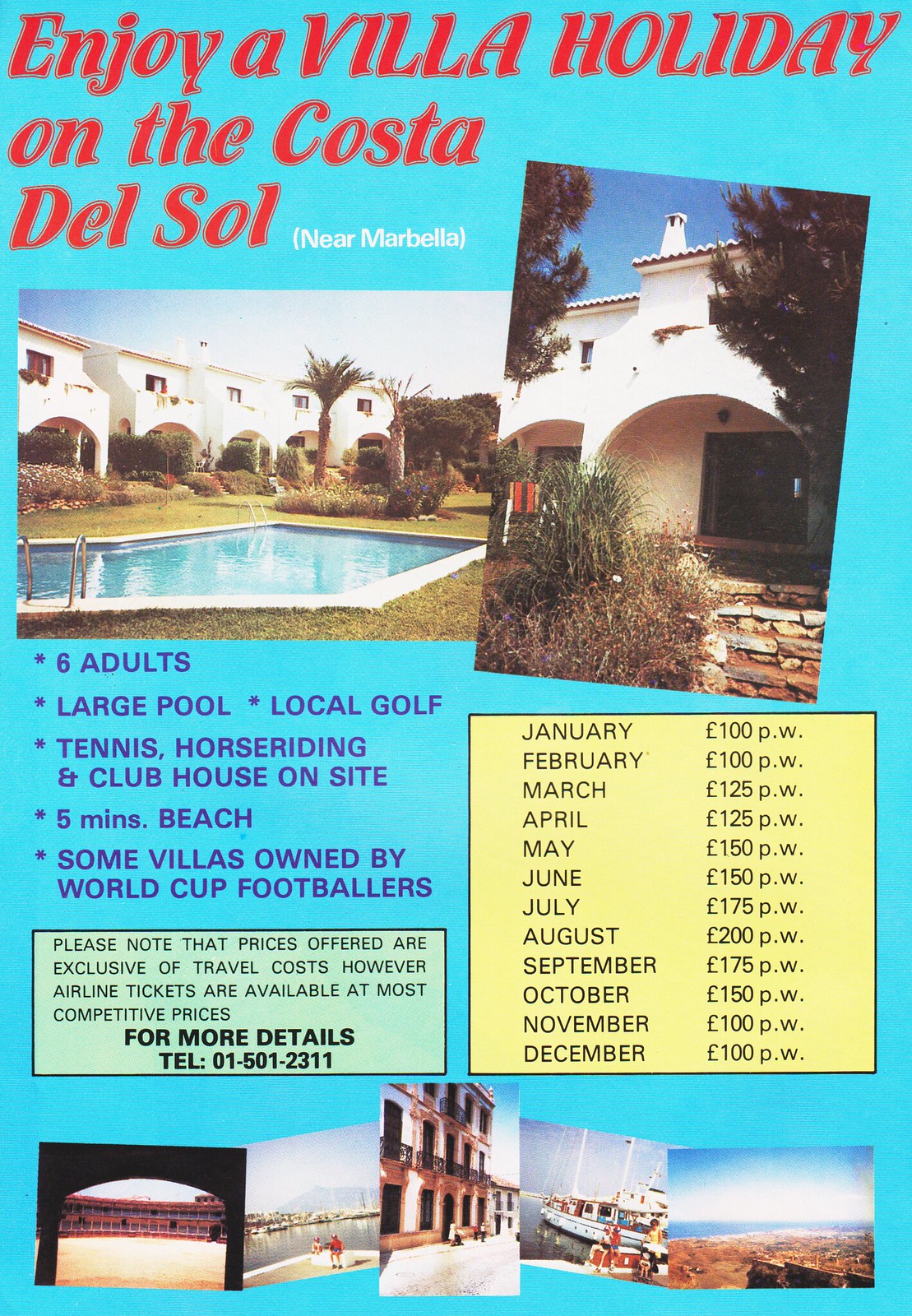Flyer advertising a luxurious villa holiday on the Costa del Sol with a light blue background. At the top, the bold red text reads "Enjoy a Villa Holiday on the Costa del Sol," while "near Marbella" is noted in smaller white font. Below the headline, two pictures showcase the resort: the left image features an expansive pool in front of square-shaped white buildings with palm trees and well-manicured landscaping. The right image is a close-up, highlighting white buildings with arches, shrubbery, and stairs.

In the middle left, blue font emphasizes key amenities: "Six adults, large pool, local golf, tennis, horse riding, and clubhouse on site." It mentions the beach being five minutes away and some villas owned by World Cup footballers.

Below, within a green rectangle, black font warns that prices are exclusive of travel costs but advises that airline tickets are offered at competitive prices. For more details, contact telephone 01-501-2311.

To the right, in a beige box with a black outline, a seasonal pricing chart displays costs ranging from $100 to $200 depending on the time of year. Further down are five additional images highlighting local landmarks, including a beach, a dock with boats, and a downtown area.